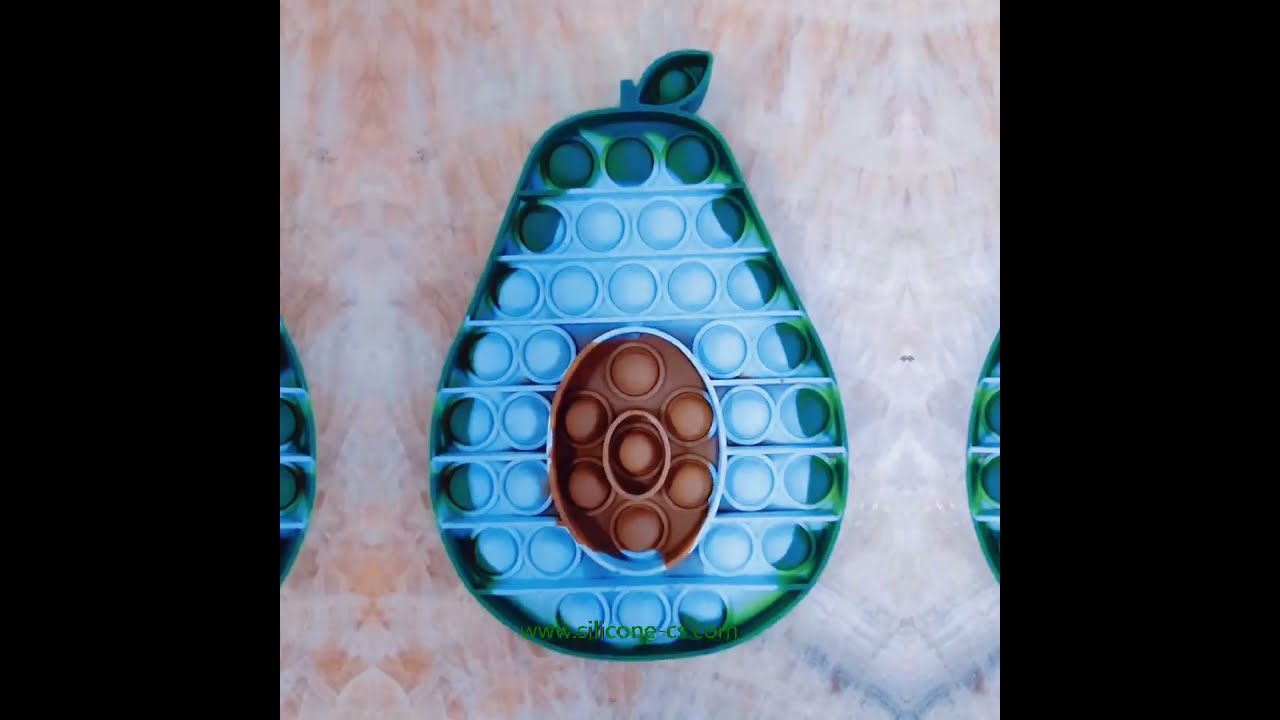The image is a digitally-created artwork featuring a pear-shaped avocado, with distinct sections of color that give it an animated and stylized appearance. The avocado is illustrated with a green outer layer transitioning to a blue interior around a prominent brown seed in the center. The composition includes intricate details, such as a small stem and a baby leaf at the top. The background exhibits a mix of pink and white hues, providing a contrasting backdrop to the vivid colors of the avocado. The image, which appears to be a cropped screenshot from a website, includes the address www.silicone-something. The scene is set against a background resembling a marble surface, with black borders on either side, suggesting it may have been presented on a table indoors. There is no additional identifying information or date provided.